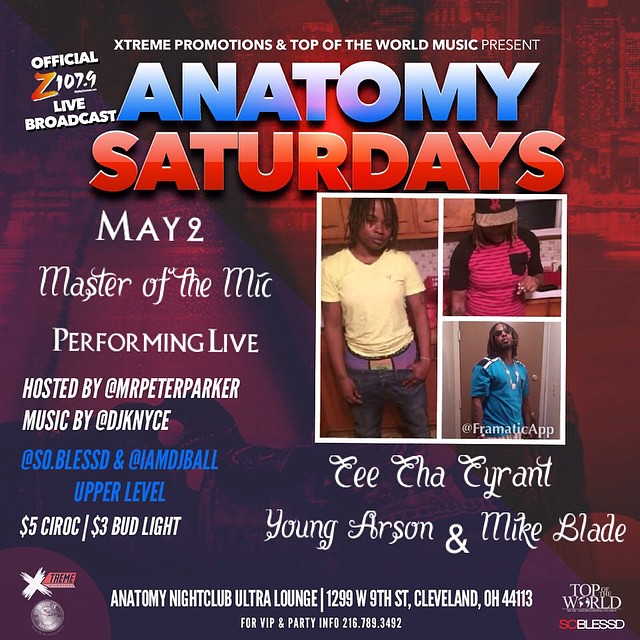The promotional poster is a vibrant square graphic advertisement with a red-to-purple gradient background. At the top, it features the text “Extreme Promotions and Top of the World Music Present” in white. Right beneath, the words "Anatomy" in large blue letters and “Saturdays” in large red letters stand out prominently. To the left, also in white text, it states “Official Z107.9 Live Broadcast” with the "Z" highlighted in orange and yellow. The event details include “May 2nd, Master of the Mic Performing Live," hosted by Mr. Peter Parker, with music by DJ K-NYCE.

Various social media handles such as @So.Blessed and @IAMDJBall are listed in blue. Drink specials, "$5 Ciroc / $3 Bud Light," are highlighted in white. The poster includes images of three African American individuals: a man with dreadlocks in a yellow shirt, another figure in a red striped shirt and ball cap, and the same individual in a blue shirt. The names C-CHA Tyrant, Young Arson, and Mike Blade are listed beneath these images.

At the bottom center, the location details are provided: “Anatomy Nightclub Ultra Lounge, 1299 West 9th Street, Cleveland, Ohio, 44113,” alongside VIP and party info with the contact number 216-789-3492. Finally, logos and additional texts, including “Top of the World” and “So Blessed,” appear in the lower corners, adding a finishing touch to this detailed and energetic poster.